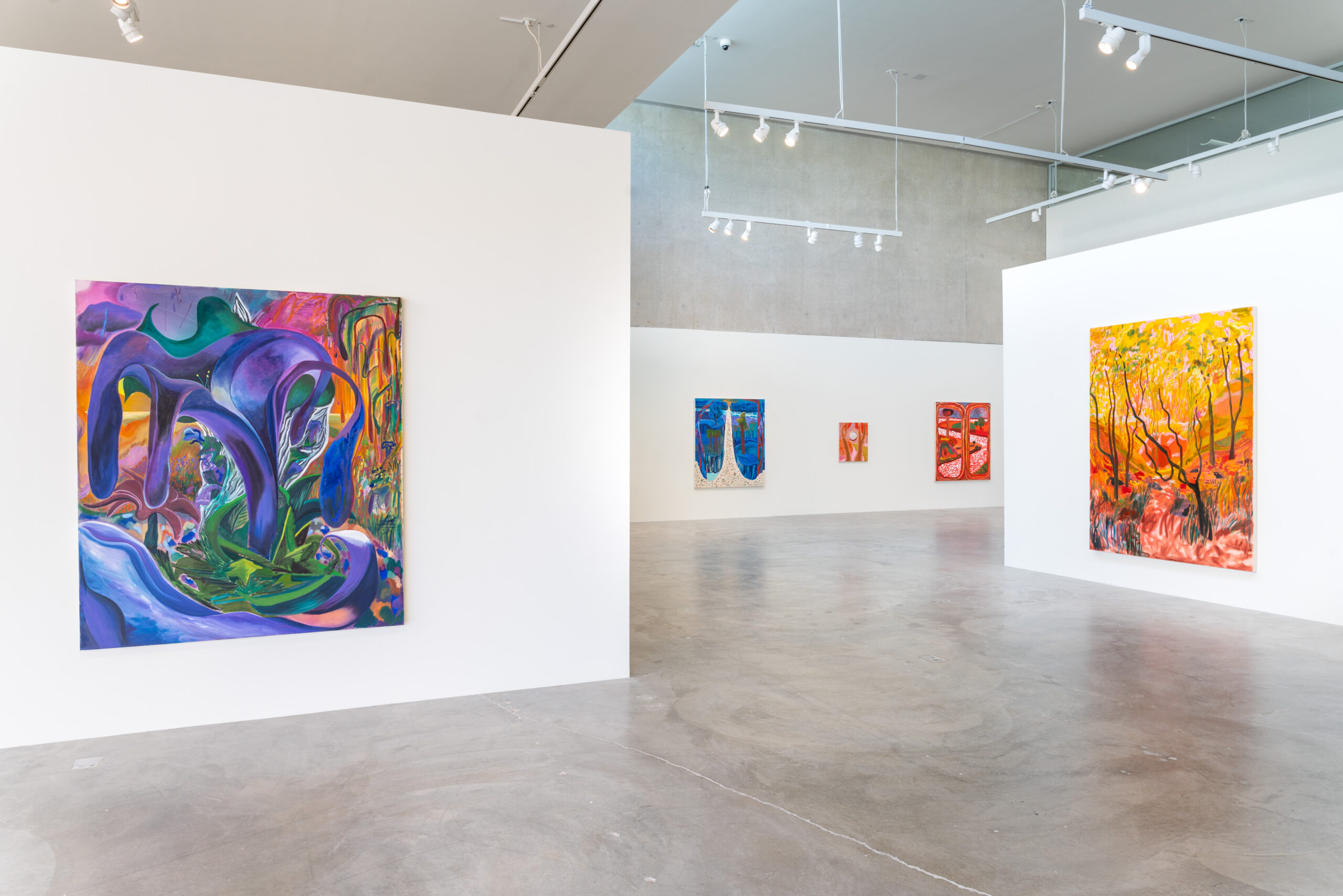This image captures the interior of an art studio, showcasing its modern, minimalist design. The studio features large white walls and a high ceiling adorned with rows of spotlights that cast a bright illumination on the exhibited paintings. The smooth, glossy concrete floor, which appears slightly reflective, enhances the spacious, airy atmosphere of the room.

Prominently displayed on the left wall, a striking square painting features purple paint flowing into a green section beneath it. On the right wall, another large canvas depicts an evocative landscape with yellow trees at the top and a creek running through it, complemented by splashes of red and white at the bottom. 

In the background, a walkway leads to yet another expansive white wall containing three more paintings. The leftmost artwork displays a yellow point rising from the middle, flanked by blue sections. Nearby hangs a smaller painting with an orange background, and to its right is another piece, also dominated by orange hues, featuring a pinkish roof with silver bars and round, yellow-lit lights hanging from long strings. The overall collection, though modern and abstract in style, seems to include both fantastical elements and landscape themes, characterized by a rich palette of vivid colors.